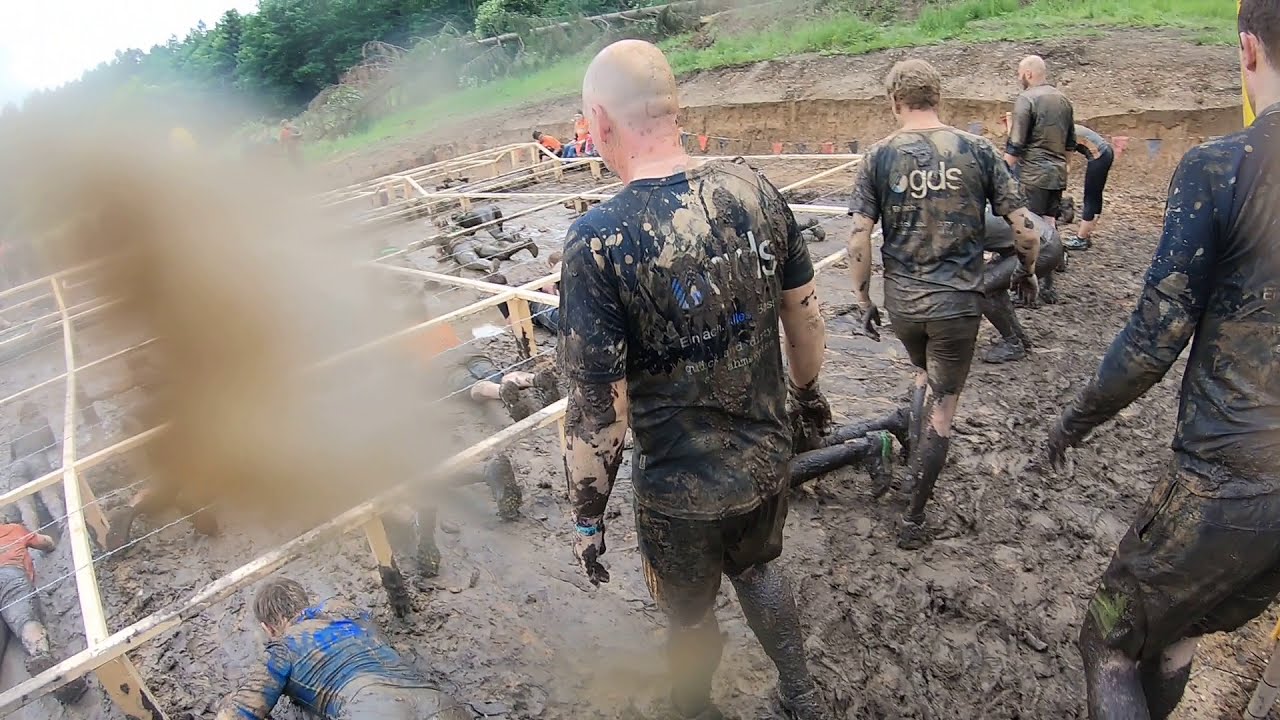This image captures an outdoor, military-style obstacle course centered around a large, dug-out mud pit, approximately two feet deep. Participants, dressed predominantly in all black with a few in blue and red shirts, are either crawling on their stomachs under a low wooden framework strung with barbed wire or preparing to do so. This part of the course requires them to stay low to avoid the barbed wire, reminiscent of battlefield training under simulated overhead gunfire. About 30 participants are actively crawling through, while roughly eight others, covered in mud, await their turn on the right side of the frame. The background features a green field bordered by pine trees, suggesting a summer setting as indicated by the participants' shorts and t-shirts. The image is partly obscured by mud splatters on the camera lens, adding to the gritty realism of the scene. The left edge of the frame is specifically streaked with mud, further intensifying the rugged environment depicted.